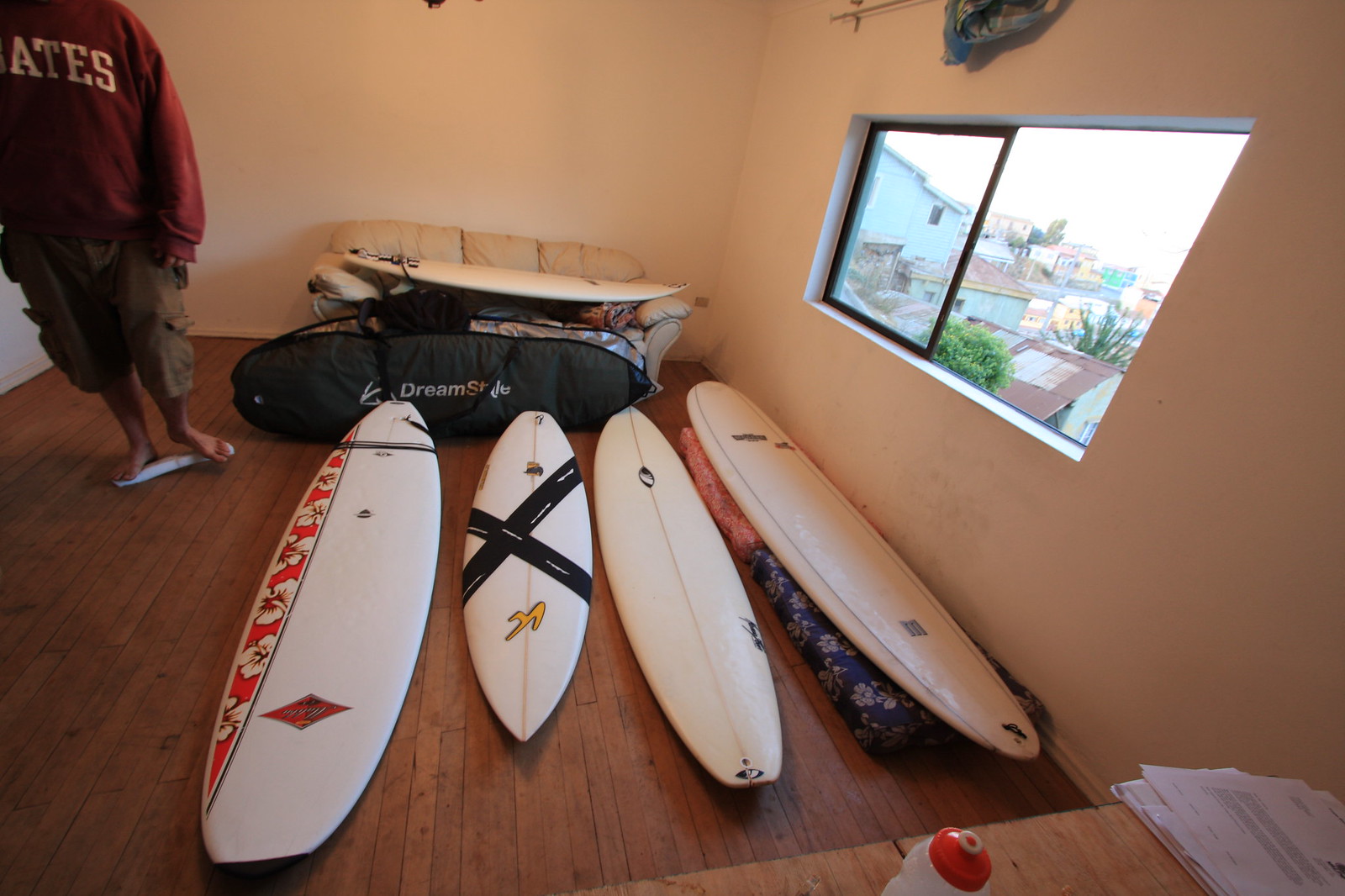The photograph captures a sparse indoor space, likely a living room or bedroom, in a beach town, evidenced by the visible palm trees and turquoise houses outside a square slider window with no curtains. The room has a deep wood brown floor and minimal furniture, primarily featuring a singular couch—described variably as white or gray—and a small beige leather loveseat. There is a desk or table with a few letters and a water bottle that has a red top and white bottom. 

Dominating the room are an assortment of surfboards in varying sizes, aligned across the right side of the space. They include a white board decorated with red Hawaiian flowers, another with a black cross, and others with simple lines and prints. One of the surfboards rests on two blankets with red and blue Hawaiian prints. 

A man stands on the left side of the image, identifiable only by his dark khaki or olive green cargo shorts, a red sweatshirt partially showing the letters "A-T-E-S," and no shoes. His face is not visible, but his tan brown skin indicates he has likely spent time outdoors. Additional items, like a bag presumably for carrying surfboards, hint at an active beach-going lifestyle. The room’s beige walls and general bareness contribute to its sparse, almost utilitarian feel, contrasted by the colorful surfboards and beach-themed items.